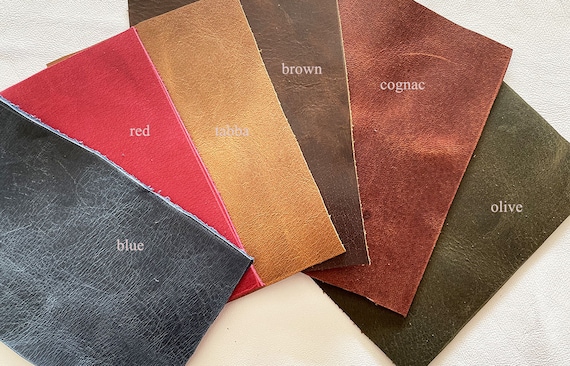The image displays six leather color samples arranged against a white background, resembling a plastic table or a white blanket. Each sample is about two inches wide by three to four inches long, featuring writing at their midpoints indicating their colors. Starting from the bottom left, the samples are fanned out like playing cards, overlapping each other. The colors, from top to bottom, are blue, red, lava (a golden brass color), brown, cognac (a brownish shade), and olive. The leather patches have a distinctive, worn texture with fine lines and veins typical of aged leather.